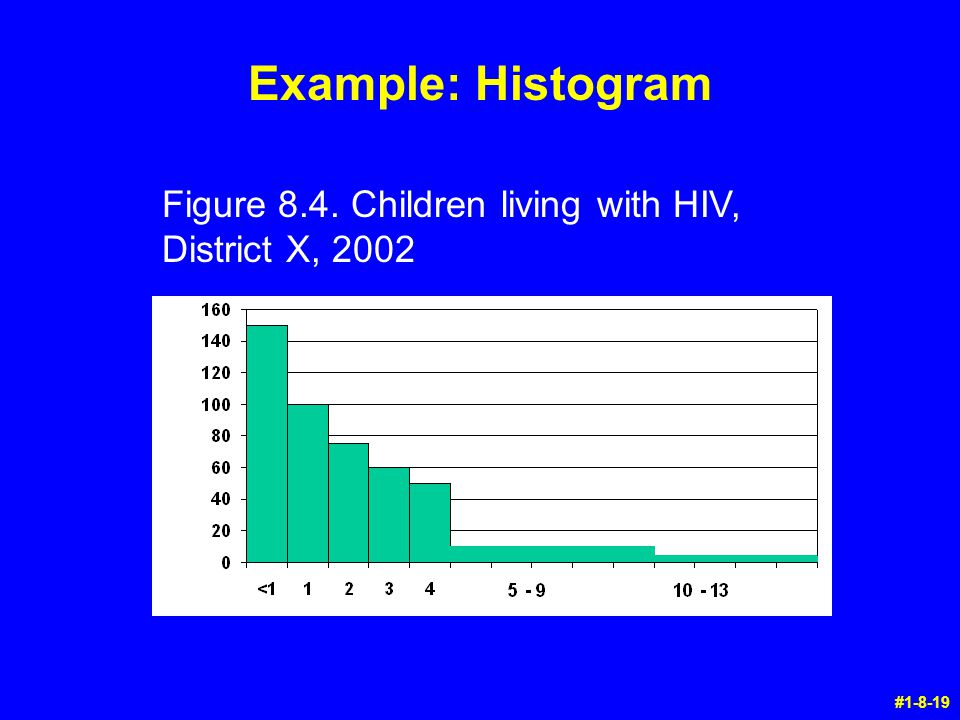The poster is a rectangular image with a stark, vibrant blue background. At the top, it features the title "Example Histogram" in bright yellow lettering, followed by text in white that reads "Figure 8.4 Children Living with HIV, District X, 2002." Below this title, a bar graph is displayed on a white background. The y-axis on the left is marked with black numbers ranging from 0 to 160 in increments of 20, and the x-axis at the bottom is labeled with categories: <1, 1-2, 2-3, 3-4, 4-5, 5-9, and 10-13. 

The bars on the graph are in a turquoise green color. The bar graph starts with the highest bar on the far left at approximately 150. Moving rightward, the bars decrease in height sequentially to about 100, 75, 60, and 50. The categories 5-9 show much smaller, roughly equal bars around the value of 10 or a little less, while the category 10-13 has the smallest bar, around the value of 5. Additionally, there is a notation in the bottom right corner in yellow letters that reads "#1-8-19". This graph effectively illustrates the decreasing number of children living with HIV in District X from highest in the youngest age group to lowest in the older age groups for the year 2002.